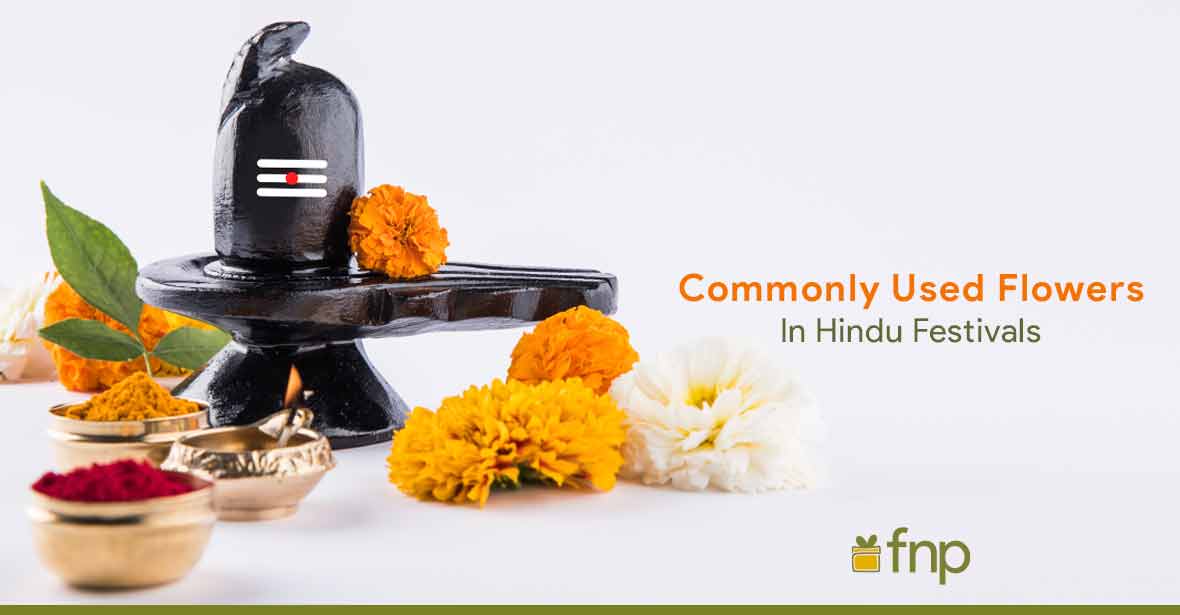This advertisement in landscape orientation features a light gray background with text overlays. In the middle to the right, the heading "commonly used flowers" appears in orange, followed by "in Hindu festivals" in green. The left side of the image is filled with various visual elements, including vibrant flowers and spices. There are prominent orange and white flowers that resemble fluffy carnations scattered around. Also present are golden bowls containing spices such as orange and red powders, adding a rich, vibrant contrast. A dark, anvil-like black table or structure occupies part of the left side, featuring three white stripes and a red dot. At its side, there's a green line stretching from the bottom left to the bottom right, intersecting with a small yellow box with a lid and two V-shaped lines. The letters "FNP" are displayed in the bottom right corner, further emphasizing the promotional aspect of the image.